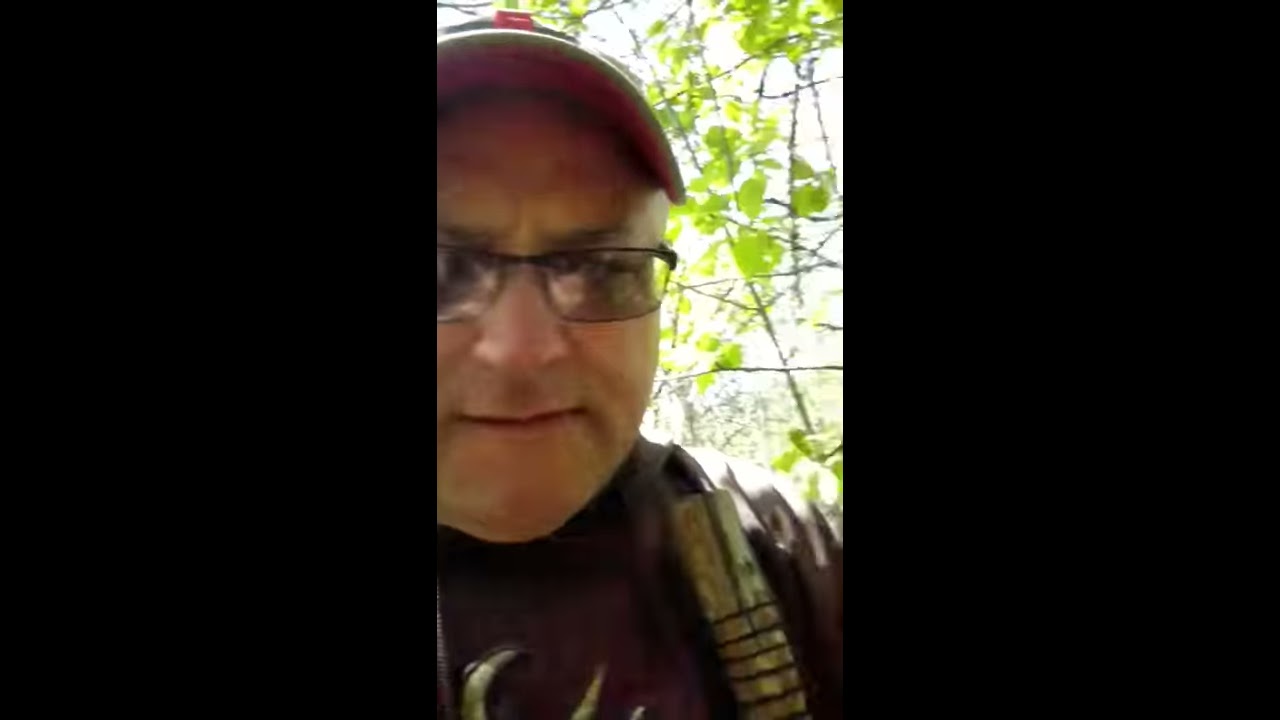The image is a photograph segmented into three vertical sections, with the left and right sections blacked out, leaving only the middle section visible. The central visible section shows a Caucasian man standing outdoors, partly in shadow and partly illuminated by sunlight. He is wearing a beige cap with a white brim and dark-framed glasses that reflect some sunlight. The man appears frustrated, his eyebrows furrowed, and his lips are thin and slightly upturned without revealing teeth. He dons a brown t-shirt that features a pattern of sharp shapes, and he has a bag with green straps slung over his shoulder. In the background, there are green tree leaves and branches, indicating he is in a leafy area. The thick black borders on either side of the image create the effect of a narrow, central slice capturing most of his face and part of his upper torso. The sunlight and tree leaves in the background add a natural, outdoor atmosphere to the photograph.